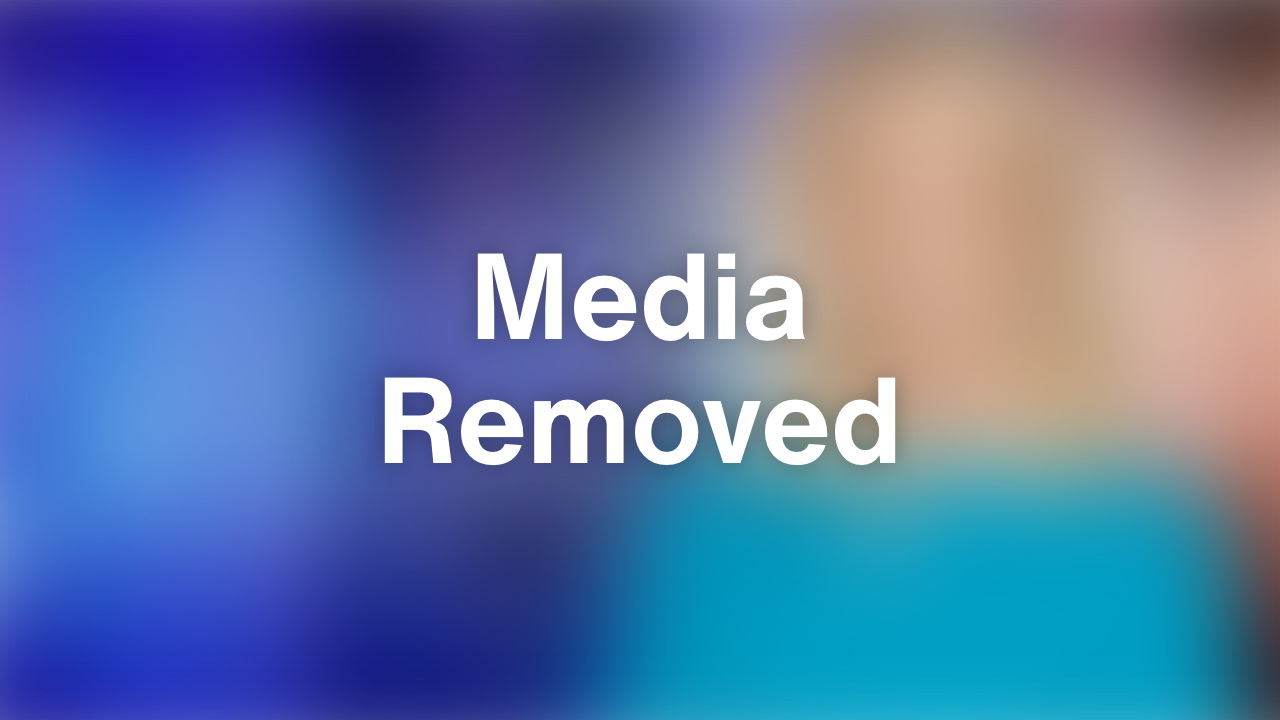This photograph captures a street artist during the daytime, working on a mural on a beige, rectangular stone wall of a building that appears to be a restaurant. The artist is depicted amidst the gloom of an overcast day, donning baggy black snow pants, dark sneakers, a gray winter jacket, green gloves, and a brown fedora-like cap. He is earnestly focused on painting a detailed mural featuring vibrant Italian ingredients: lush green basil leaves, succulent red tomato slices, and a white piece of fresh mozzarella cheese. At his feet lies an array of gray cylindrical spray paint cans, and a yellow "caution" sign can be seen in the bottom left corner of the image. The mural artist is positioned on a paved parking lot with the street visible to his right, and another beige building stands in the background under the gray sky. Additionally, an old vent is located on the bottom left of the building wall, hinting at its potential use as a restaurant.